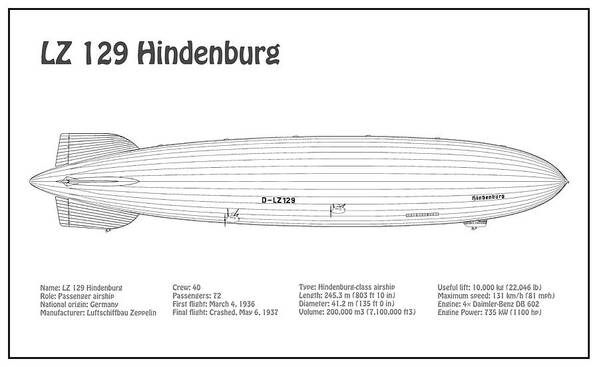The image depicts a detailed black and white sketch of the LZ-129 Hindenburg, a renowned German passenger airship. The sketch offers a computer-digitized view of the airship, akin to a technical drawing or blueprint. Clear text on the top left corner labels the airship as "LZ-129 Hindenburg." Additional information is presented below the sketch, stating the airship's name, role as a passenger airship, and its German origin. The manufacturer is specified as Luftschifferbau Zeppelin. Key specifications include a crew capacity of 40, passenger capacity of 72, a first flight date of March 4th, 1936, and a crash date of May 6th, 1937. The airship is classified as a Hindenburg-class airship, with a length of 245.3 meters, a diameter of 41.2 meters, and a volume of 200,000 cubic meters. Its useful lift is 10,000 kilograms, maximum speed is 131 kilometers per hour, and it is powered by four Daimler-Benz engines producing a total of 735 kilowatts. The overall image is clearly visible, with the setting brightened by proper lighting, ensuring that all details are easily discernible.